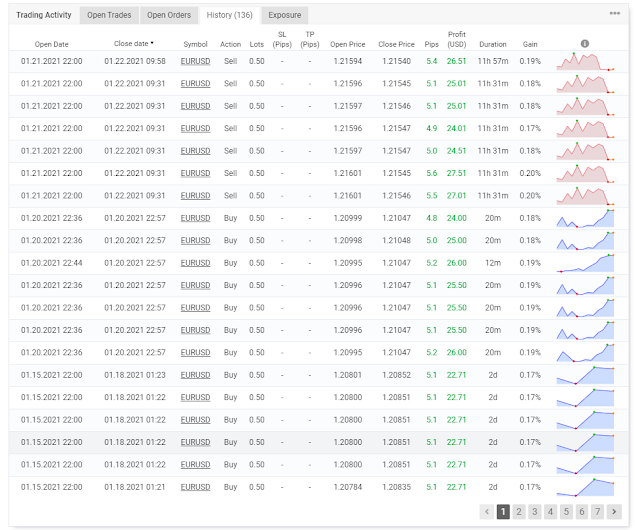The image displays a detailed webpage related to trading activities, filled with numerous data points at first glance. At the top of the page, there are tabs labeled "Trading Activity," "Open Trades," "Open Orders," "History," and "Exposure." These tabs are in gray bars, except for the "History" tab, which has a parenthetical note indicating (136).

The main content of the webpage is structured in a tabular format with multiple columns. The first column is titled "Open Date" and lists dates and times vertically. The second column, "Closed Date," similarly displays dates and times. The following column, "Symbol," indicates trading pairs, specifically "EUR/USD" (Euro/US Dollar).

Next, the "Action" column specifies whether the trade involved buying or selling. The "Lots" column quantifies the number of lots traded. The columns labeled "SL Pips" and "TP Pips" likely denote stop-loss and take-profit points in pips, respectively. The "Open Price" and "Closed Price" columns provide the prices at the opening and closing of trades.

Additional columns include "PIP," which shows numerical values often highlighted in green, and "Profit (USD)," which displays profit figures in US dollars. The "Total Profit" column accumulates overall profits, and "Duration" indicates the length of each trade in hours or minutes. The "Gain" column shows percentages, representing the profit or loss from each trade.

A graphical representation is present at the top of the table, depicting the performance of the top five or six trades with a line graph. The lines of the graph are red at the top and blue below, each dotted periodically. Pagination at the bottom of the table indicates the presence of multiple pages, specifically seven in total.

Overall, the dense and organized layout captures a comprehensive record of trading activities, readily providing an array of data points for detailed analysis.